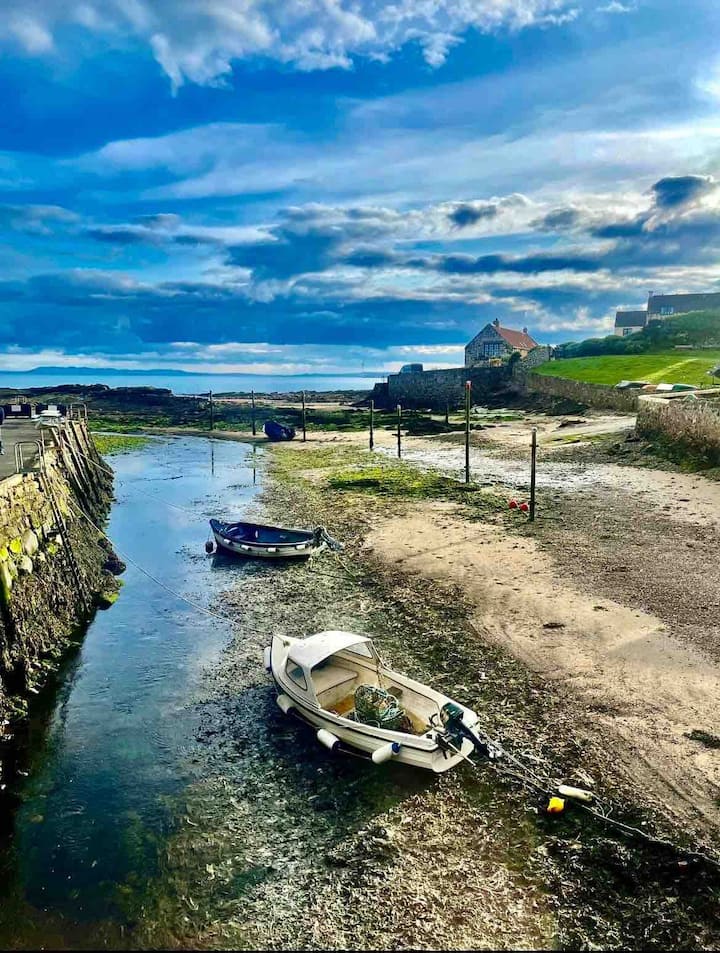In this striking photograph, a collection of boats rests on a dry, muddy riverbank, indicating a dramatic drop in water levels that has transformed what used to be a viable waterway into a mere stream. The boats, including an old white boat with a motor and a rowboat, are tethered by ropes to long-forgotten docks. The backdrop reveals rolling green hills with houses perched on cliff tops, some encircled by brick fences. The bright blue sky, interspersed with large, dramatic clouds, sets a vivid contrast against the earthy tones below. In the distance, you can make out the shimmering ocean, hinting at the river's former connection to it. Features such as scattered posts stuck in the ground and ladders leading up small cliffs add to the scene’s sense of desolation. Apart from the patches of dark green grass, the landscape appears somewhat barren, with a dusty road and a parking lot-like area near what appears to be a murky beach. This melancholic image captures the essence of an old fishing village or town grappling with the fading remnants of its once-thriving waterways.